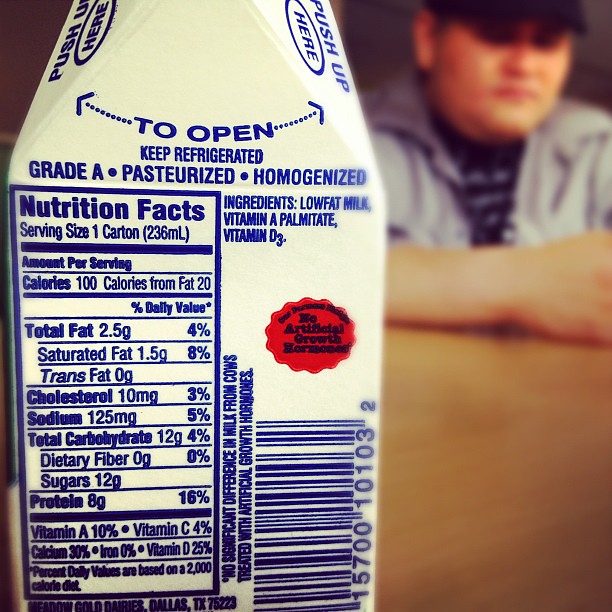The image features a close-up view of a white milk carton with dark blue lettering and a noticeable red sticker reading "no artificial growth hormone or hormones." The carton is prominently displayed on the left side of the photograph, showcasing detailed nutritional information and ingredients: "Keep refrigerated, Grade A, pasteurized, homogenized, low-fat milk, vitamin A palmitate, vitamin D3." It lists nutrition facts for a serving size of one carton (236 milliliters), with 100 calories per serving, 20 of which are from fat, including 4% of the daily recommended total fat, 8% of daily saturated fat, zero trans fats, 3% of daily cholesterol, 5% of daily sodium, 4% of daily carbohydrates with 12 grams of sugar, and 16% of daily recommended protein. The carton is open, though the top lip is cut off from the frame.

In the background, a slightly blurred figure appears, possibly a young male wearing a black hat and a gray shirt with a collar. He seems to be seated at a table, which varies in description from light brown to white wooden. The person is resting their hands on the table, potentially holding a phone, adding a casual atmosphere to the scene, reminiscent of a typical lunch setting.